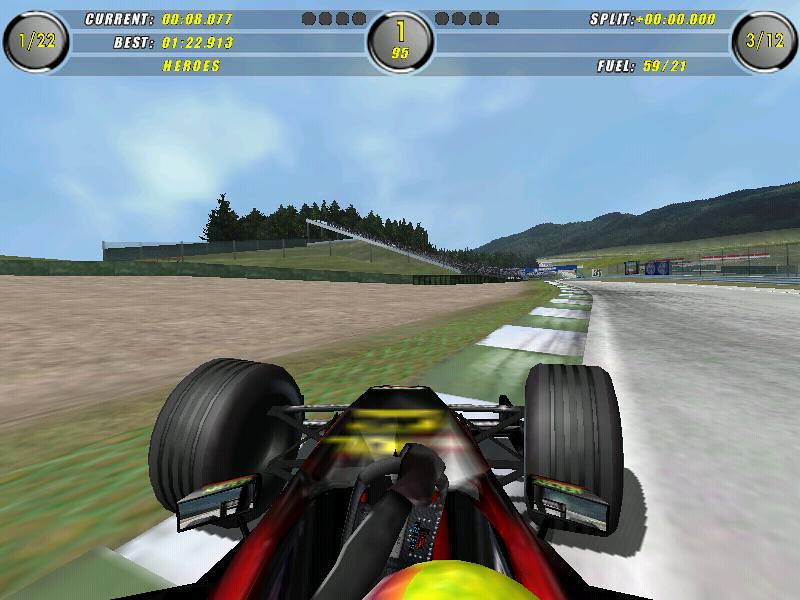The image depicts a video game screen showcasing the front end of a sleek formula-style race car, characterized by its exposed wheels, which extend beyond the narrow, aerodynamic, rocket-shaped body. The race car is primarily black adorned with striking yellow and red accents. The oblong-shaped racing steering wheel, seen partially, features a black and gray color scheme with silver rivets. The driver's helmet, barely visible at the bottom of the image, is a vivid combination of yellow and orange. He appears to be wearing a dark racing suit with black and gray gloves. The car is positioned on the left side of the racetrack, navigating a turn closely hugging the white line marking the edge. The scenery includes distant hills and trees under a clear, bright blue sky with minimal cloud cover. On the left side of the car lies a dirt field, while to the right, the smooth paved surface of the racetrack is visible.